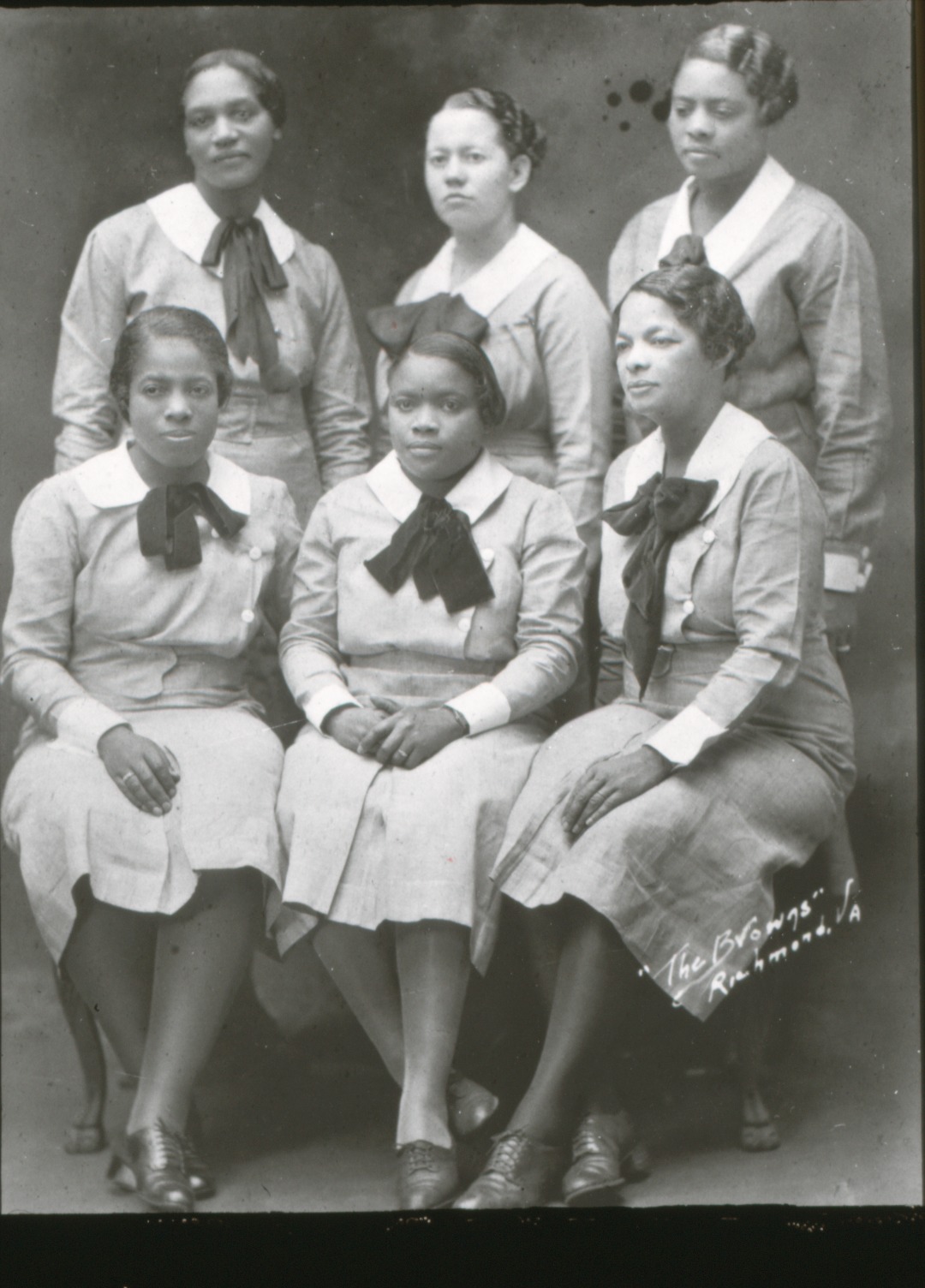This black-and-white photograph, possibly from the 1940s or 1950s, features six African-American women posing stoically for the camera. Three women are seated on chairs or a bench in the front, while three others stand behind them. They are all in their 20s and wear matching uniforms—a tan dress or skirt outfit with prominent white collars and thick black ribbon ties, reminiscent of what French artists might have worn. Their hairstyles, pulled back in various ripply styles, add a touch of individuality amid their coordinated attire. Despite the degraded quality of the image, their poised and formal expressions stand out. Handwritten text at the bottom of the image reads "The Brownies," suggesting they might be a musical group. Additional text indicates a connection to "Richmond, Virginia."